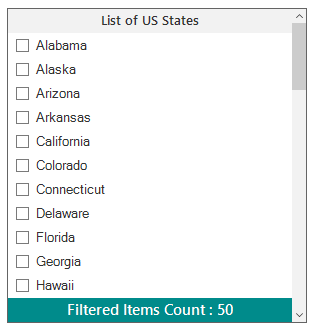This image displays a small, white background square with a list of U.S. states and corresponding checkboxes. There are a total of eleven checkboxes, each aligned with a state name in a vertical column. The states listed next to each checkbox are as follows in order: Alabama, Alaska, Arizona, Arkansas, California, Colorado, Connecticut, Delaware, Florida, Georgia, and Hawaii. 

Below the list, there is a label that reads "Filtered items count" followed by the number 50, suggesting that the list is part of a filtered search or selection. On the right side of the square, there is a scrollbar, positioned at the top, indicating that there are additional states and checkboxes visible upon scrolling down. The rest of the background outside this square is plain and empty.